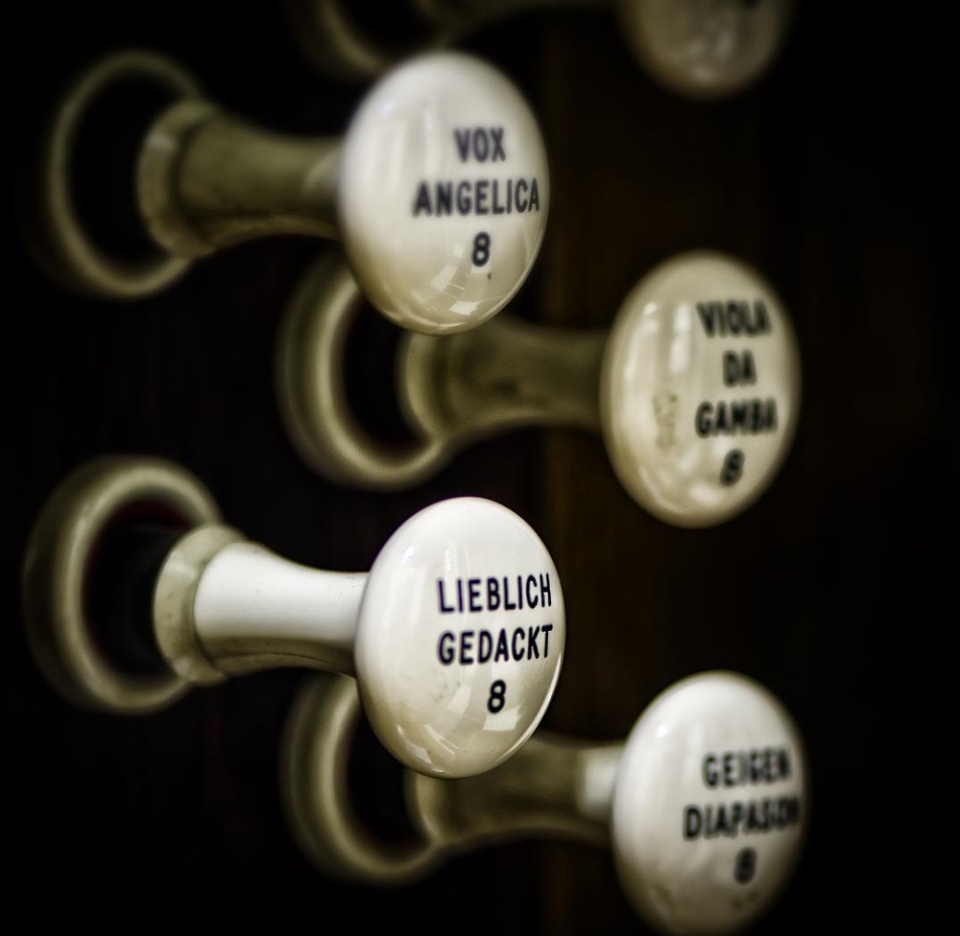This image features a series of four prominent, glossy white knobs protruding from a black surface on the left side. The knobs are uniformly cylindrical, with a lustrous finish, resembling ceramic material. They evoke a sense of precision and craftsmanship, reminiscent of chess pieces due to their refined contours. Each knob is set into silver-coloured sockets embedded within the black wall, providing a striking contrast to the shining white of the knobs.

Starting from the top, the first knob is labeled "Vox Angelica" in crisp black text, with the number "8" positioned below it. Directly underneath, the second knob bears the name "Viola da Gamba" with the number "8" following. This particular label appears slightly blurred, affecting its legibility. The third knob is inscribed with "Lieblich Gedacht," accompanied by the number "8" beneath it, maintaining clarity in its text. The final visible knob, similar to the second one, has a slightly unclear label, possibly reading "Gedger" or a similar term, with the second line starting with the letter "D." Additionally, the edge of what seems to be another knob is just visible at the very top of the image, suggesting a fifth knob might be partially out of frame.